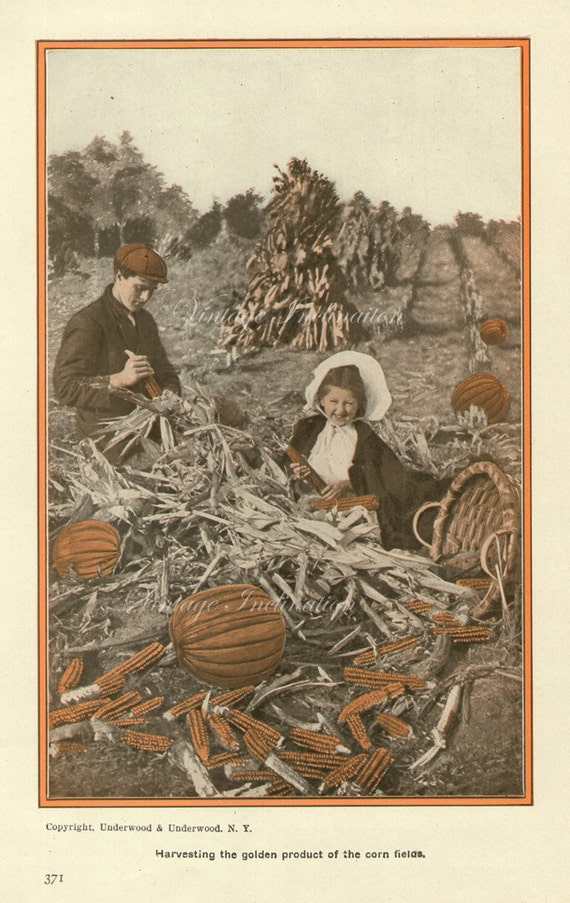This appears to be a page from an old book or magazine, characterized by a yellowed, off-white background. The page is numbered 371 on the lower left. The centerpiece is a portrait-oriented, colorized sepia-toned photograph with an orange hue, depicting a nostalgic autumn farm scene. The image features a boy and a girl harvesting corn and pumpkins in a hay field, amidst a setting evocative of Thanksgiving. The boy, positioned slightly left, sports a proto-baseball hat with a short brim and is engaged in shucking corn. To his right is a girl wearing a white bonnet, holding a piece of orange-colored corn, evocative of a pilgrim outfit. In front of them lies a heap of corn husks, shucked corn, and scattered pumpkins, all notably tinted in shades of orange and brown. The photograph bears the text at the bottom: "Harvesting the Golden Product of the Cornfields," and is credited to "Copyright Underwood and Underwood, New York."